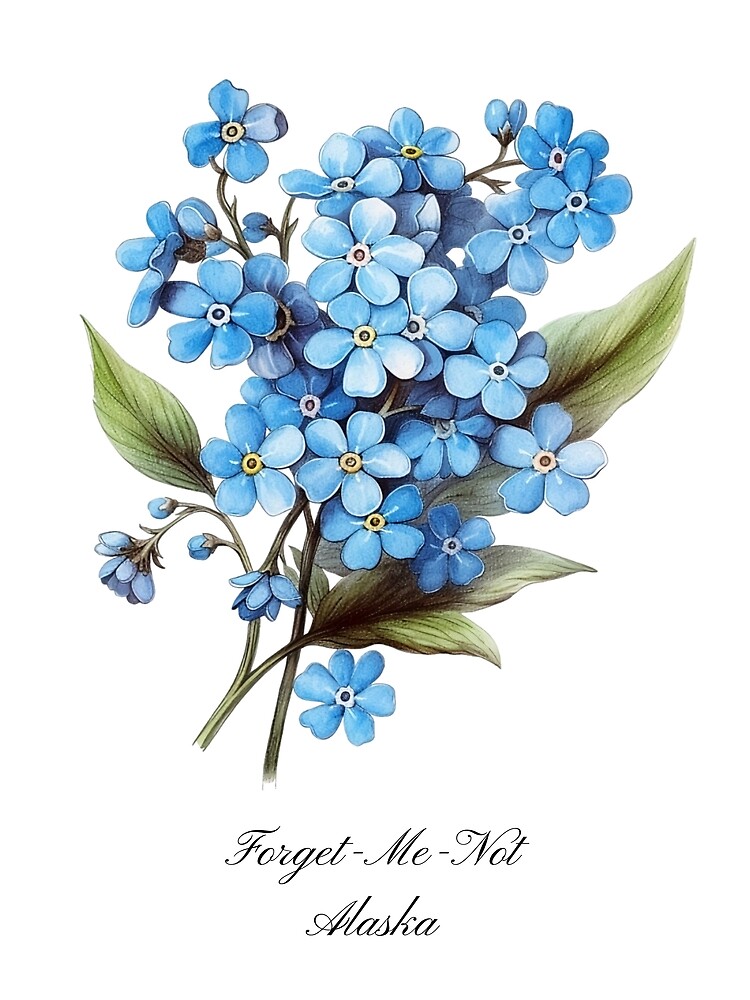This illustration features an artistic representation of Forget-Me-Not flowers, drawn against a pure white background. The flowers prominently display their signature five light blue petals, with their centers varying between yellow and white hues. The foliage consists of five to six green leaves, sprouting from two main green stems, which branch out in multiple sections, though some branches are obscured by the dense floral arrangement. The image exudes a delicate, almost clip-art style, reminiscent of designs found on greeting cards or seed packets. At the bottom, in elegant cursive script, the text "Forget-Me-Not Alaska" is written, with each word starting with a capital letter. The minimalistic yet detailed depiction emphasizes the beauty and simplicity of these iconic flowers, set against a stark white backdrop that enhances the vivid colors and intricate details of the illustration.